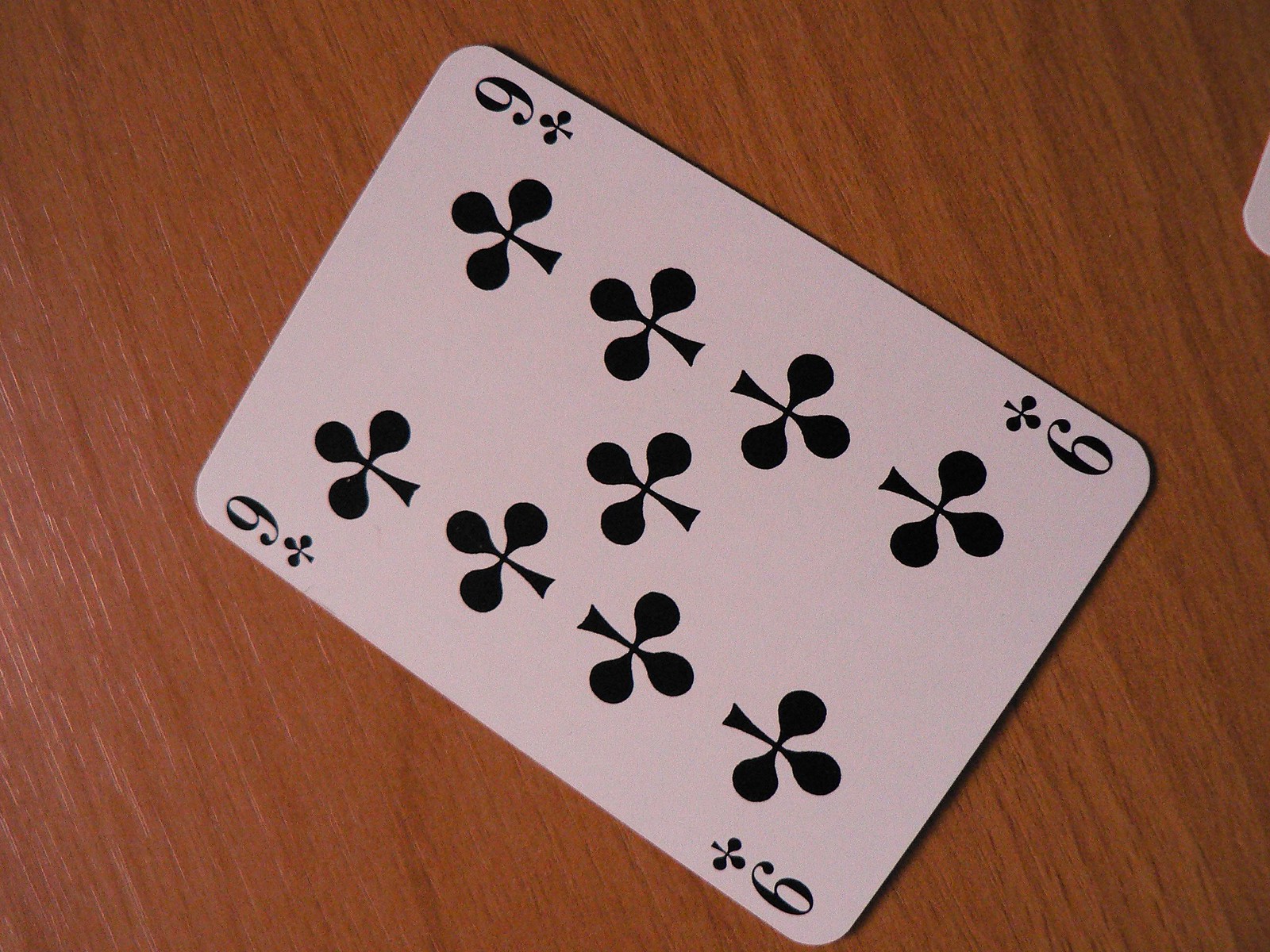This image features a nine of clubs playing card, predominantly white with black symbols. Each corner of the card displays a small, black "9" and club symbol. The arrangement of the clubs on the card is symmetrical: four clusters on each side with a single club in the center. When viewing the card from one direction, five clubs are upright, while four clubs appear upside down when viewed from the opposite direction. The card rests on a wooden surface with visible scratches, adding texture and character to the background.